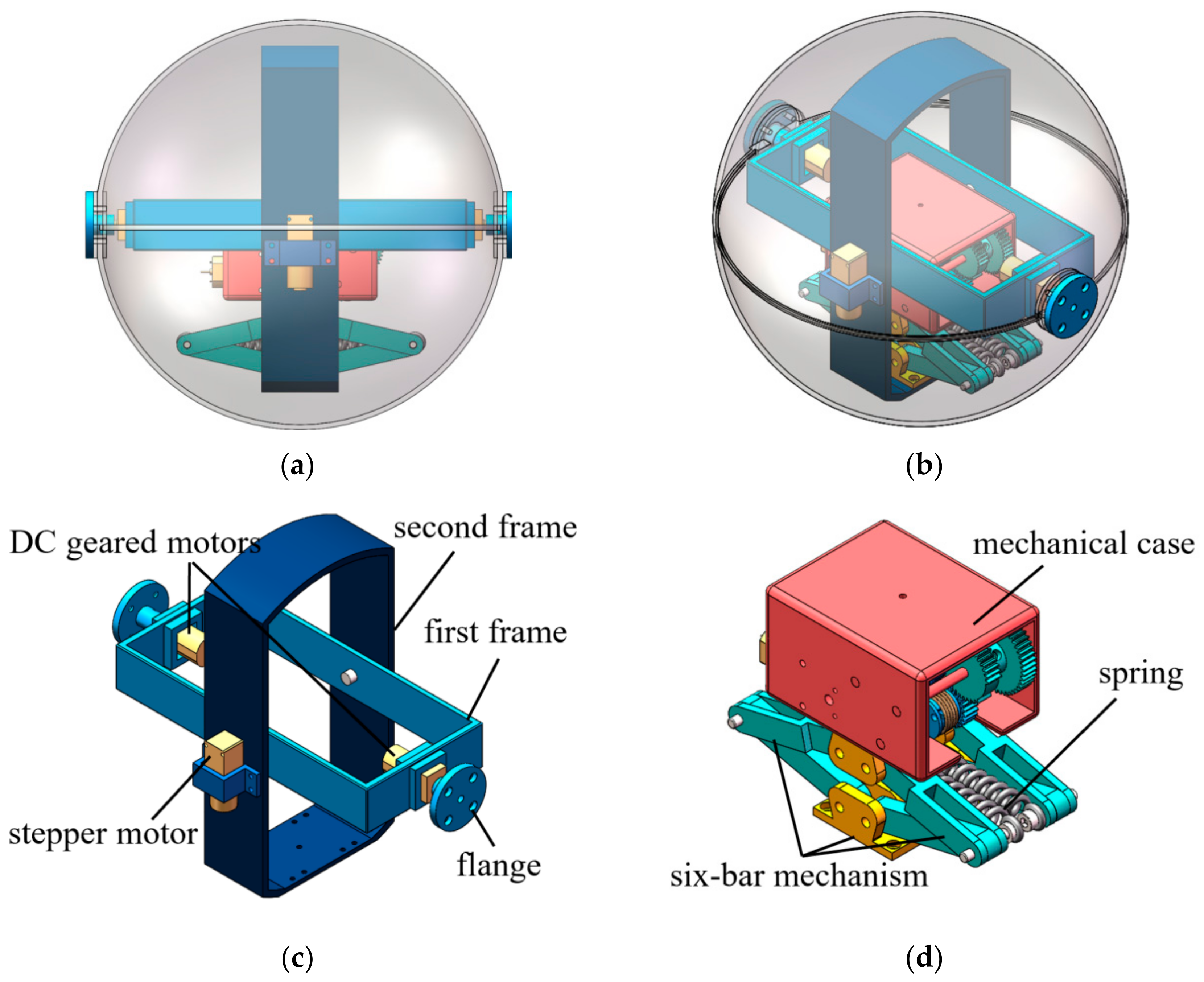The image is a detailed four-part diagram labeled A, B, C, and D, illustrating the inner and outer components of a mechanical gadget. Parts A and B are encased in a glass dome with two distinct blue screws on either side of the dome. Inside the dome, a rounded top metal gadget visible in Part A shows the front of this mechanism, while Part B focuses on the top view. Part C provides an in-depth look at the labeled internal frame components of the gadget, detailing things such as the DC geared motor, first and second frames, stepper motor, and flange. Part D, with a white background, uncovers the intricate inner workings of the gadget, featuring a red case, teal legs, and a yellow base supported by labeled components including the mechanical case, springs, and a six-bar mechanism. All diagrams are meticulously labeled with black writing, providing a comprehensive overview of the gadget’s configuration.